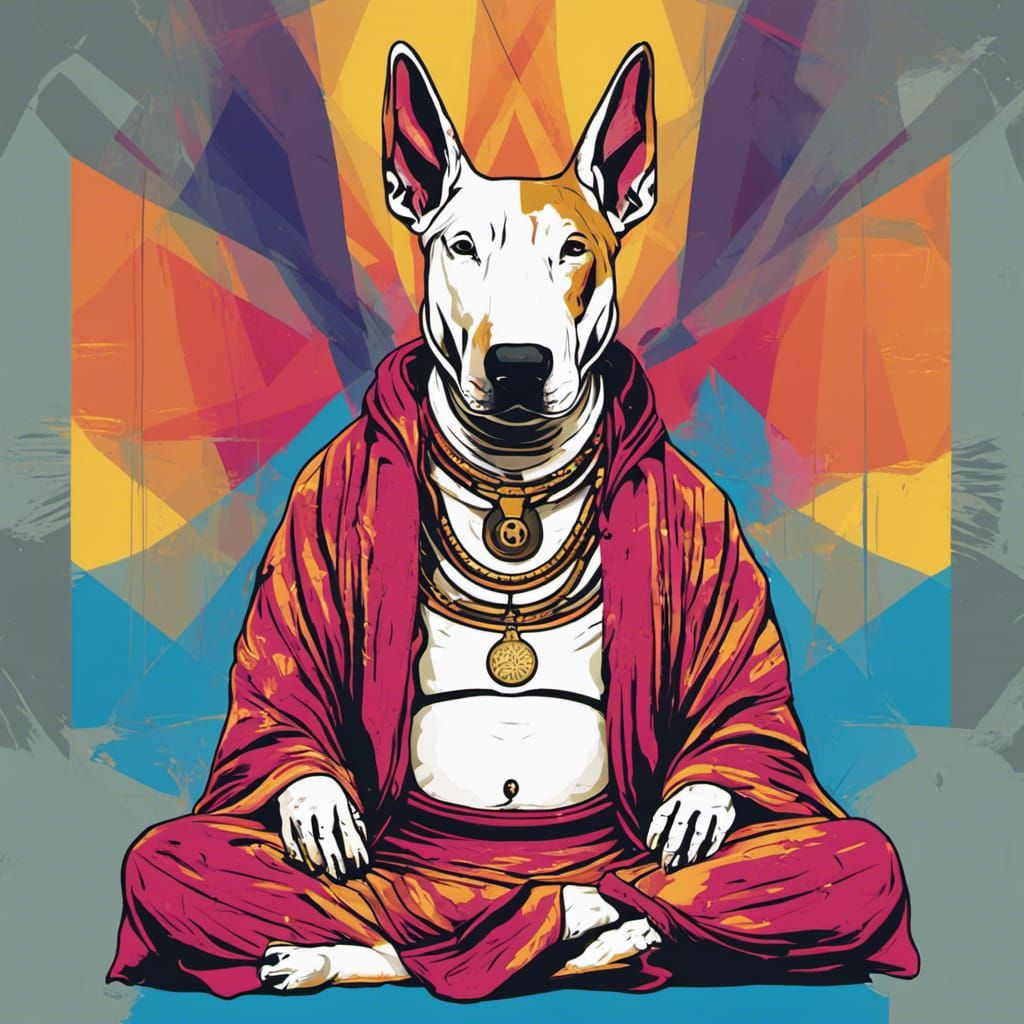The image features a cartoon-like illustration of a dog with anthropomorphic characteristics, rendered in a style reminiscent of cel-shaded animation or an Andy Warhol-inspired painting. The dog, which has a body predominantly white in color, exhibits a mix of human and canine features. It has human-like knees and fingers, yet retains its canine paws, which have black claws. 

Sitting cross-legged, the dog is dressed in baggy red pants and a similarly oversized red hoodie that is unzipped, revealing a large pot belly and chest. Adorning its neck are multiple gold chains with round pendants. The dog’s head, resembling that of a Great Dane, has a distinct brown spot around its right eye, pointed ears with red inner linings, and a black nose. 

The background is a vivid tapestry of colors—gray, light and dark purple, orange, yellow, pink, red, light blue—arranged in a variegated pattern that adds to the image’s dynamic and lively aesthetic. The setting against this colorful backdrop merges the whimsical nature of the illustration with the vibrant complexity reminiscent of modern pop art.